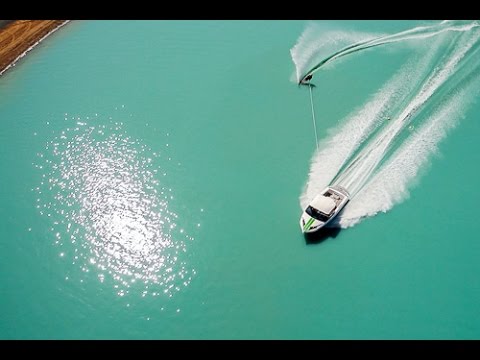This overhead image captures a scene of a vibrant, blue water body with a white speedboat slicing through the calm expanse. The boat, adorned with two green racing stripes along its center, creates dynamic patterns in the water with its swift movement, leaving a trail of frothy, white waves in its wake. To the right of the boat, a person is seen wakeboarding, carving their own path and adding their distinct wave patterns to the scene. The sun's reflection on the water is striking, casting a dazzling, almost white glare on the left side of the image. The serene surroundings feature a sandy shoreline visible at the top left, marked with faint tire tracks indicating recent activity. This juxtaposition of the boat's vigorous pace against the tranquil, smooth water, framed by natural reflections and the distant shore, creates a captivating and detailed snapshot of aquatic adventure.